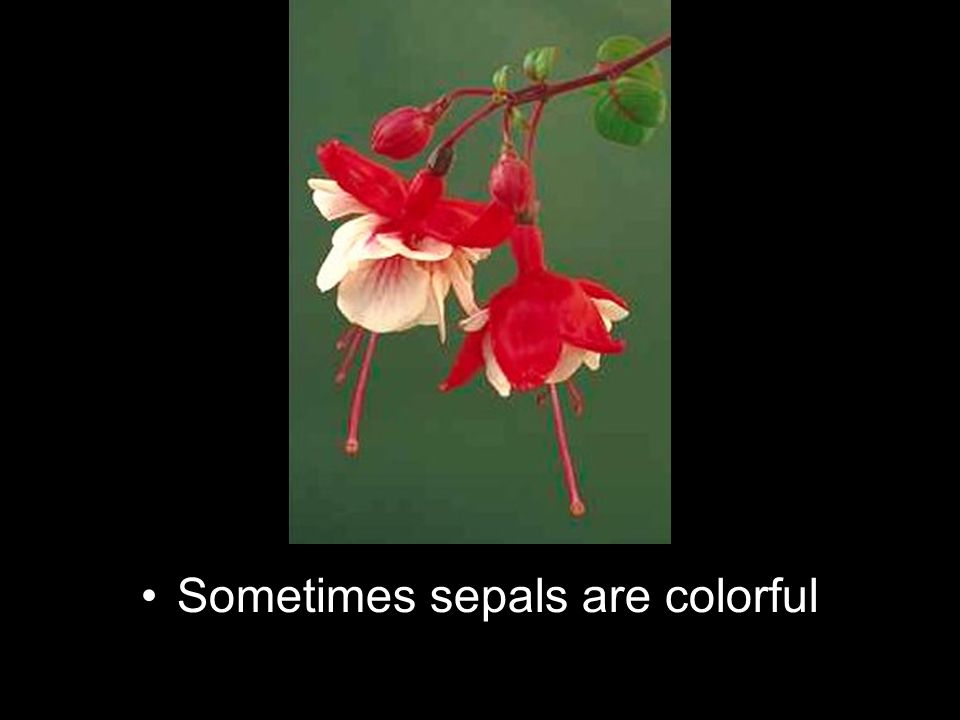This image features a close-up view of a flowering plant against a black background, with the focal point centered near the top. The plant exhibits a harmonious blend of colors, comprising green leaves and a combination of red and white blossoms. There are two prominent flowers, each emerging from the branch of a tree. Surrounding these flowers are green leaves that perfectly round out the scene.

The flowers start as small, striking red buds before blossoming into their full beauty. As they bloom, the outer red petals open to reveal inner white petals, creating a layered effect reminiscent of a tiny dancer wearing a tutu. Long red stamens protrude gracefully from the center of each flower, ending in tiny balls, adding to the elegant appearance.

Beneath this botanical display, in the black background, is a bullet-pointed line of white text. The text reads, "Sometimes sepals are colorful," with an uppercase "S" starting the sentence. This caption elucidates that the vibrantly colored parts of the flowers being observed might indeed be sepals instead of petals, showcasing the natural beauty often attributed to these unique structures.